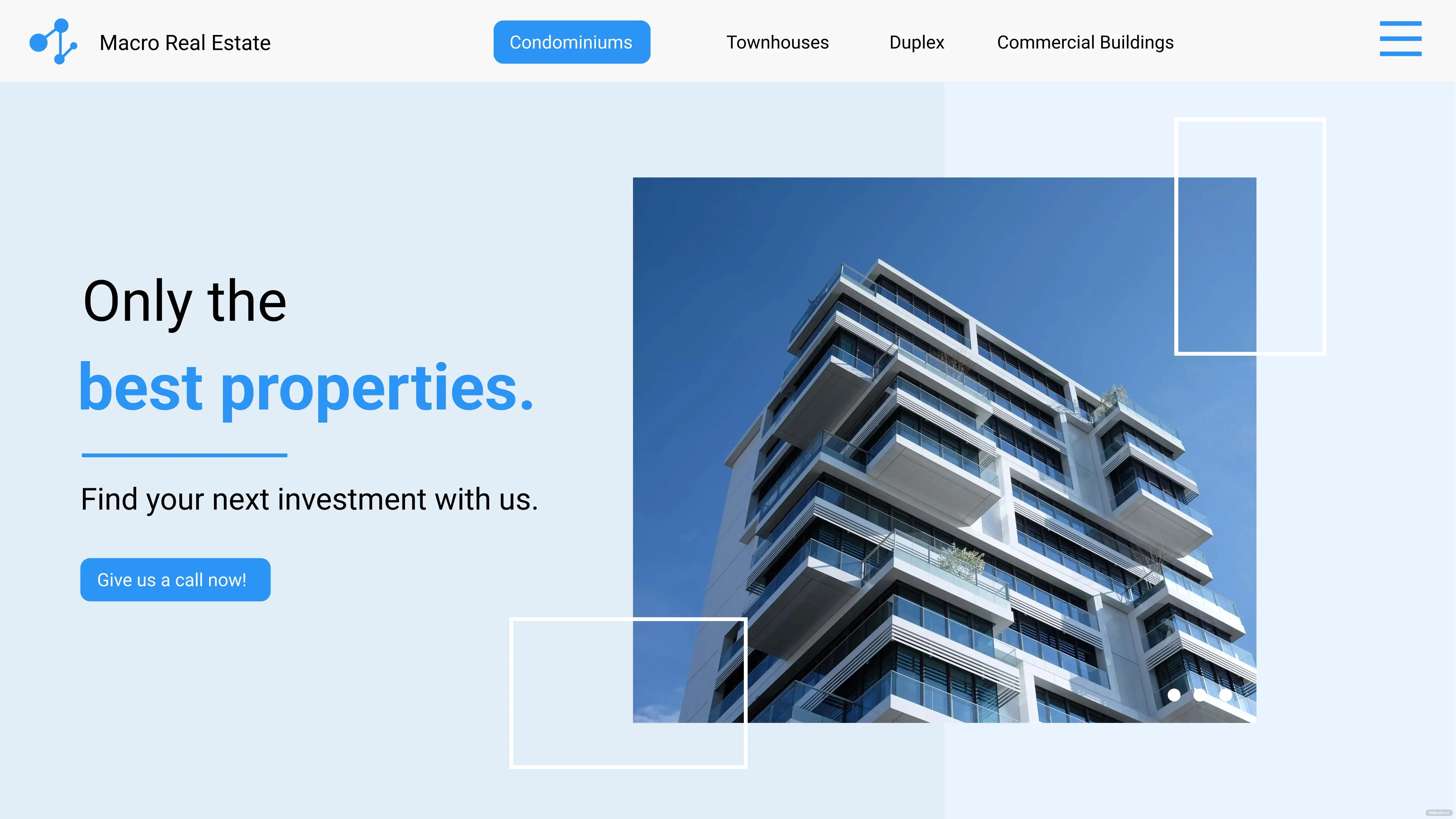This image appears to be a screenshot from a real estate website displayed on a computer screen. The background is predominantly a light blue color. On the right side of the screen, there's an image framed by a gray border at the top. Inside this section, there's a blue line ending in blue dots, with another smaller blue dot on a black line branching off. The heading "Macro Real Estate" is prominently displayed.

Below the heading, there are navigation options listed vertically: Condominiums, Townhouses, Duplex, and Commercial Buildings. The "Condominiums" option is highlighted in blue, indicating it is the selected category. On the far right side of the screen, three vertical lines are aligned in a column.

The central part of the image features a light blue background on the left side with the text "Only the Best Properties. Find your next investment with us." prominently displayed. Below this text, a blue rectangular button invites users to "Give Us a Call Now." The phrase "Best Properties" is emphasized in blue, underlined by a blue line.

To the right of this text, there's a graphic depicting a large apartment building with numerous windows and balconies. The building is set against a blue sky. Additionally, there are two white rectangles, one in the lower left corner and one in the upper right corner of this graphic.